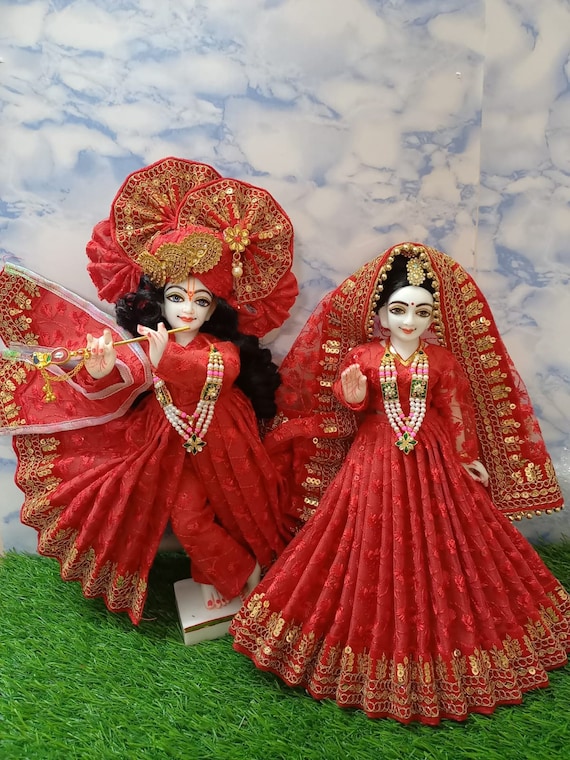In this portrait-mode image, we are presented with two intricately detailed dolls standing on realistic-looking grass with a backdrop painted to resemble a blue sky adorned with fluffy clouds. Both dolls are dressed in elaborate red gowns with gold accents and intricate bead necklaces made up of three thick strands. The doll on the right features a vibrant red headdress that cascades past her waist, while the doll on the left sports an extravagant headdress resembling several gold-adorned fans stacked together, creating a striking, tall silhouette. Additionally, this doll is depicted playing a metallic flute-like instrument, adding an artistic touch to the scene. The dolls' white faces and black hair, complemented by bendy dots between their eyebrows, highlight their Asian-inspired design, enriching the cultural authenticity and visual appeal of the display.